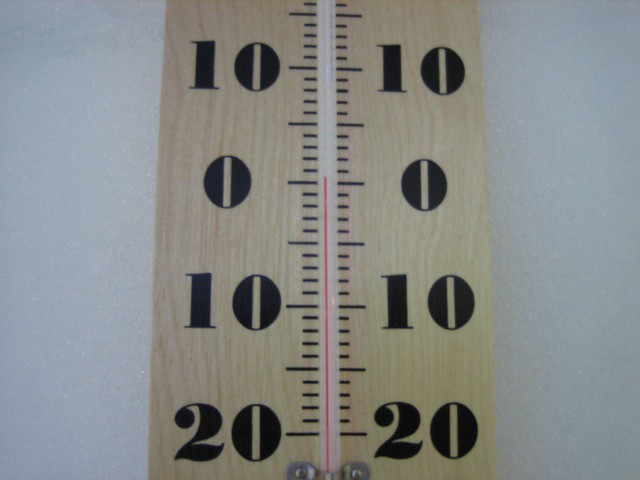This is a detailed close-up image of a wall thermometer, zoomed in for precise inspection. The thermometer appears to be propped against a backdrop of white-painted drywall, though it's not clear if it is mounted or simply leaning. The thermometer casing is constructed to mimic wood, though it is uncertain if it's genuine wood or a faux material. The visible segments of the thermometer display measurements from -10 to 20 degrees, with these markers appearing on both the left and right sides. Between each main numerical indicator, there are several smaller dashes. Each main number (such as 10, 0, 10, and 20) is marked by a thicker horizontal dash, followed by a series of thinner dashes leading to the next significant marker. The mercury column in the thermometer is currently positioned around the zero-degree mark, indicating the temperature.